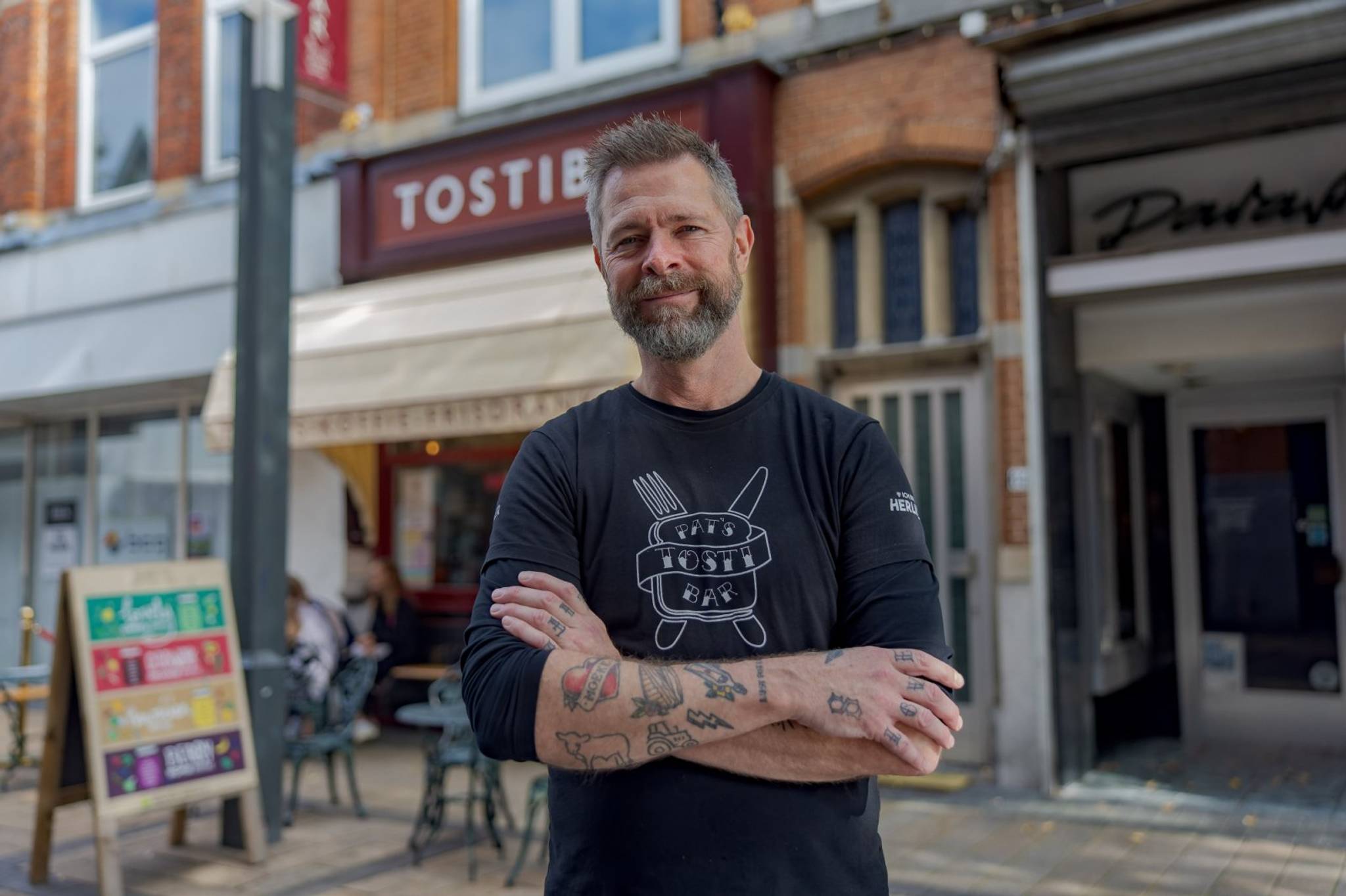A photograph captures a middle-aged Caucasian man with a short gray beard and gray hair on the sides, accented by brown hair on top, looking directly at the camera with his arms folded. He is wearing a long-sleeved black T-shirt with the sleeves pushed up to his elbows, prominently featuring a white logo that reads "Pat's Toasty Bar" alongside a fork and knife crossing through toast. His exposed arms and fingers exhibit various tattoos. The backdrop includes a bustling downtown retail district with several storefronts, likely housing shops and restaurants. Notable elements in the scene include a wooden sign on the sidewalk, seemingly advertising lunch specials, and a collection of green-colored steel tables and chairs positioned for outdoor dining. The urban setting suggests an active street life.